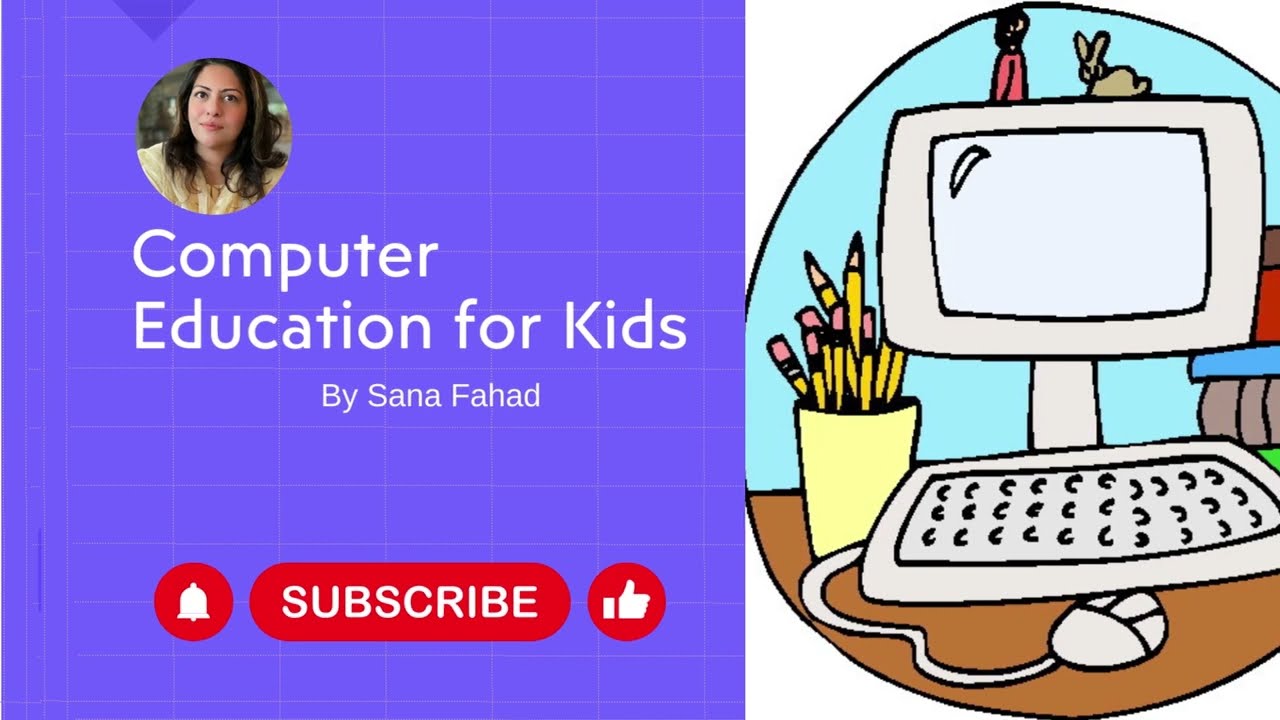The image is divided into two distinct sections. The left section features a light purple box with a pattern of white rectangles. In the upper left corner of the box, there is a circular photo of a woman with dark hair and features. Below the photo, text in white reads "Computer Education for Kids" followed by "by Sana Fahad." At the bottom of this section, there is a red bar with three elements: a bell icon on the left, a long button labeled "subscribe" in the middle, and a thumbs-up icon on the right, all resembling YouTube's notification and subscription prompts.

The right section of the image showcases an egg- or oval-shaped outline containing a childlike, retro-style drawing reminiscent of 90s clip art. This drawing includes a computer, keyboard, and mouse all placed on a brown table. To the left of the computer is a cup filled with pencils, while the right side shows a chair with a red back, blue seat, and grey legs, as well as a stack of books. Atop the computer monitor, there are two small figures: a rabbit and what appears to be a person. The computer screen itself displays a half crescent moon in the upper left-hand corner.